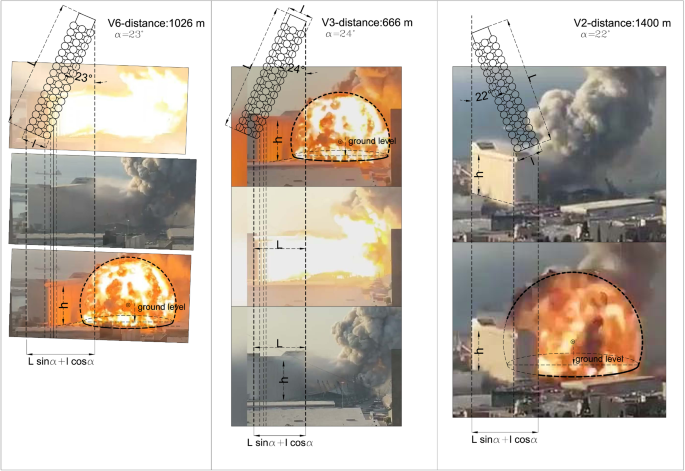This image is divided into three sections, each depicting various aspects of a single explosion from different angles, accompanied by scientific and mathematical diagrams. The left section features a vertical image labeled "V6 minus distance 1026 M" and "A equals 23," showing sky and clouds. The middle section includes three stacked photographs of smoky clouds, labeled "V3 minus distance 666 M." The right section displays two smoke-filled images marked "V2 minus distance 1400 M." Each section incorporates mathematical equations and diagrams, indicating an analysis of the explosion's dynamics and possibly the effectiveness or likelihood of extinguishing the fire. The detailed layouts suggest a comprehensive study of the explosion's impact and the subsequent smoke, though the nature of the suppression method remains unclear.